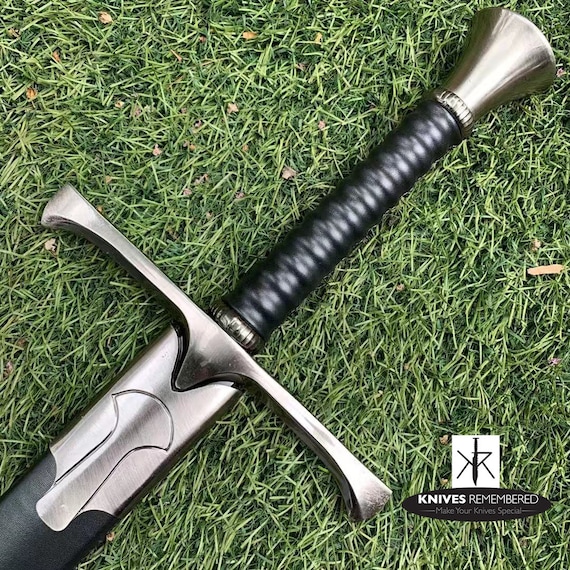In this professional daytime photograph, a sword, partially sheathed, lies diagonally on a backdrop of flattened, green grass. The sword features a long, black, ribbed handle that tapers into a sleek, metallic cone at the end. The hilt, made of brushed steel, extends horizontally, adding a sturdy aesthetic to the weapon. The sheath, which is adorned with silver engravings and a contrasting black section, obscures the blade. Dominating the lower right corner is a black oval logo with white text reading "Knives Remembered: Make Your Knives Special," suggesting this image is an advertisement for a custom knife service. The colors in the composition—black, white, gray, silver, brown, and abundant green—draw attention to the texture and craftsmanship against the natural grassy background. While the entire length of the sword isn't visible, the detailed depiction of the handle and sheath gives a clear idea of its design.